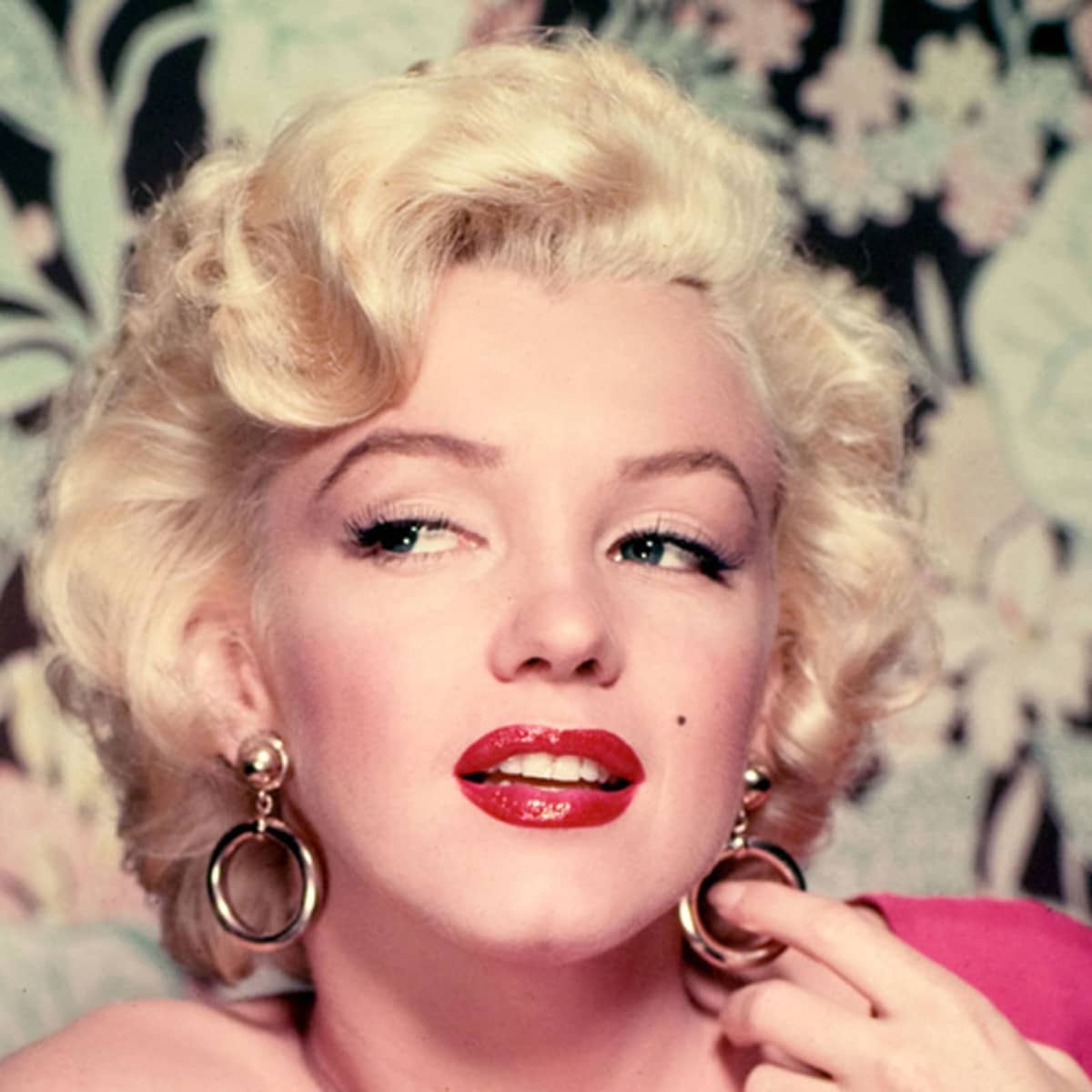In this classic color photograph of iconic film actress Marilyn Monroe, she is captured in her trademark style with short, wavy, blonde hair styled in a permed bob. Marilyn, with her fair skin and bright blue eyes, is looking off to the left of the image, her eyes slightly averted from the camera. Her makeup is meticulously done, with long eyelashes and bold, ruby red lipstick that highlights her slightly parted lips, revealing her top teeth and adding a touch of allure. A single mole adorns the side of her right cheek, enhancing her distinctive beauty.

Marilyn is dressed in a pink top, one side casually draping off her shoulder. Adding to her glamorous look are large, gold hoop earrings, and her left index finger is playfully hooked inside the hoop of the earring in her left ear. The background is blurred but features a black canvas adorned with pink and white flowers that beautifully complement her attire and makeup, emphasizing her timeless elegance. The photograph perfectly captures Marilyn's iconic image, with an expression that seems to be a poised yet candid glimpse of the star in a moment of classic Hollywood grace.